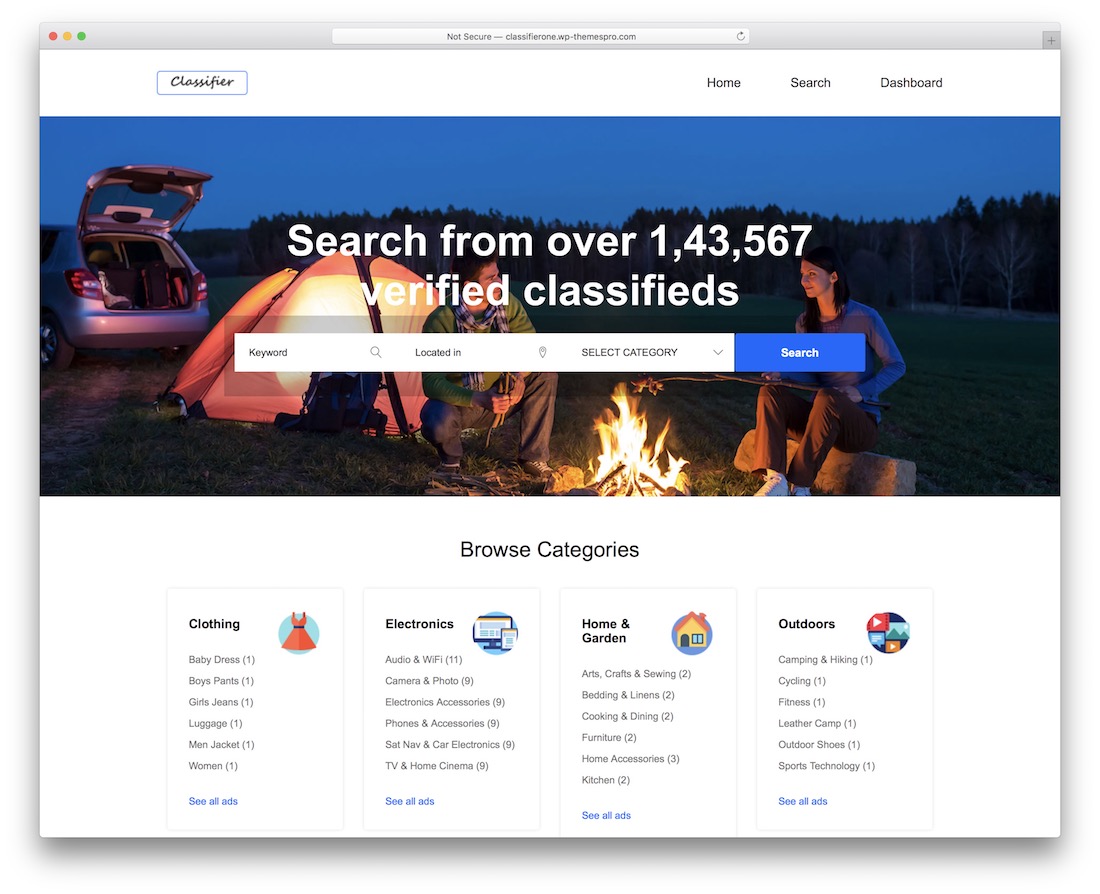**Image Caption:**

At the top of the image, there is a header indicating "Not Secure" accompanied by three circles: red, yellow, and green. On the top left, the word "Classifier" is displayed, while the top right includes options for "Home," "Search," and "Dashboard."

Below the header, the image captures a picturesque outdoor scene set in a field during dawn or dusk. In the foreground, a car with its trunk open is visible. Adjacent to the car, there is a tent and a campfire, around which a man and woman are roasting marshmallows. This conveys a serene camping experience.

In the middle section of the image, there's a text stating "Search for over 1,435,567 verified classified." Below this, there is a search box where users can input keywords, select a category, and initiate a search.

Further down, there is a section labeled "Browse Categories" featuring four boxes. Each box is labeled with an icon and a category: "Clothing," "Electronics," "Home and Garden," and "Outdoors." Each category also contains additional links for more specific subcategories or options.